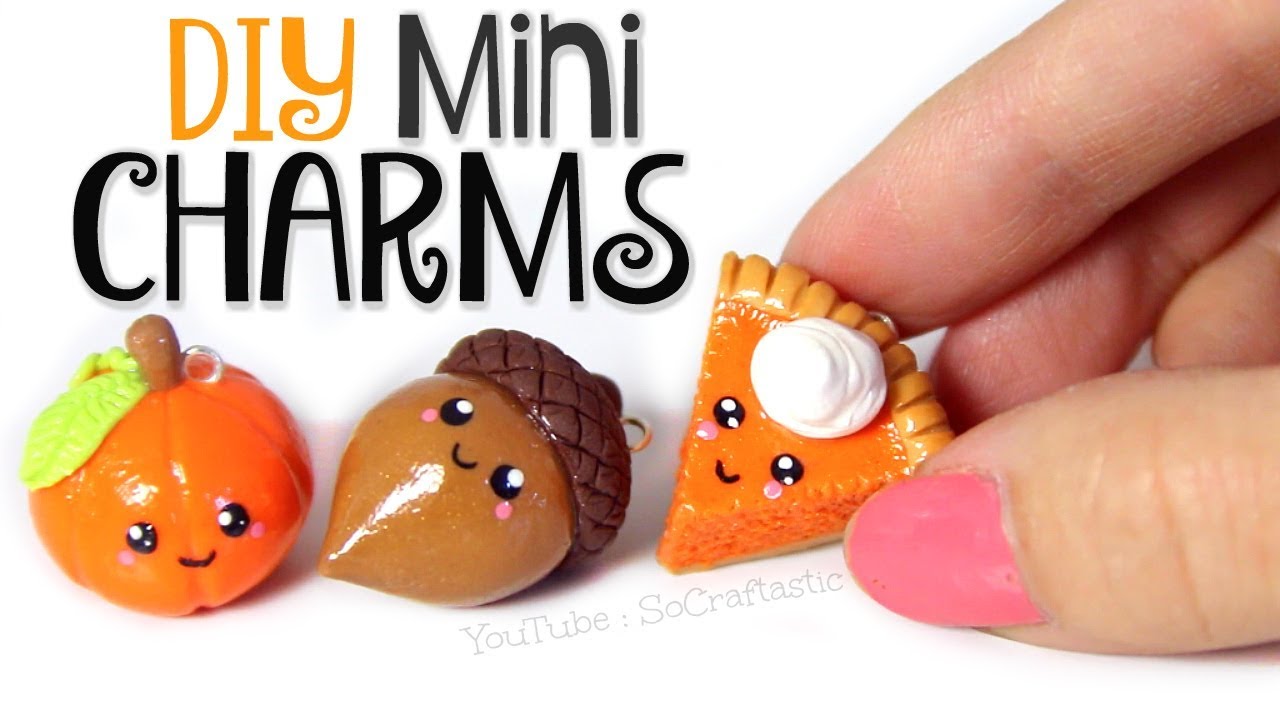The image is a banner graphic titled "DIY Mini Charms," with "DIY" in yellow and "Mini Charms" in black written in a fun, curly font at the top left. Beneath the title text, there are three adorably crafted charms arranged from left to right: the first is a small pumpkin with a green leaf, a smiley face, and a tiny hole for attaching keychains or keyrings. The second charm is an acorn with a brown top, black eyes, pink accents under the eyes, and a light brown bottom, also with a smiley face. The third charm is a piece of pumpkin pie with whipped cream on top and a smiley face, held delicately by a woman's hand with pink fingernail polish on her thumb and first finger. Below the charms, there's a small gray watermark that reads, "YouTube SoCraftastic."